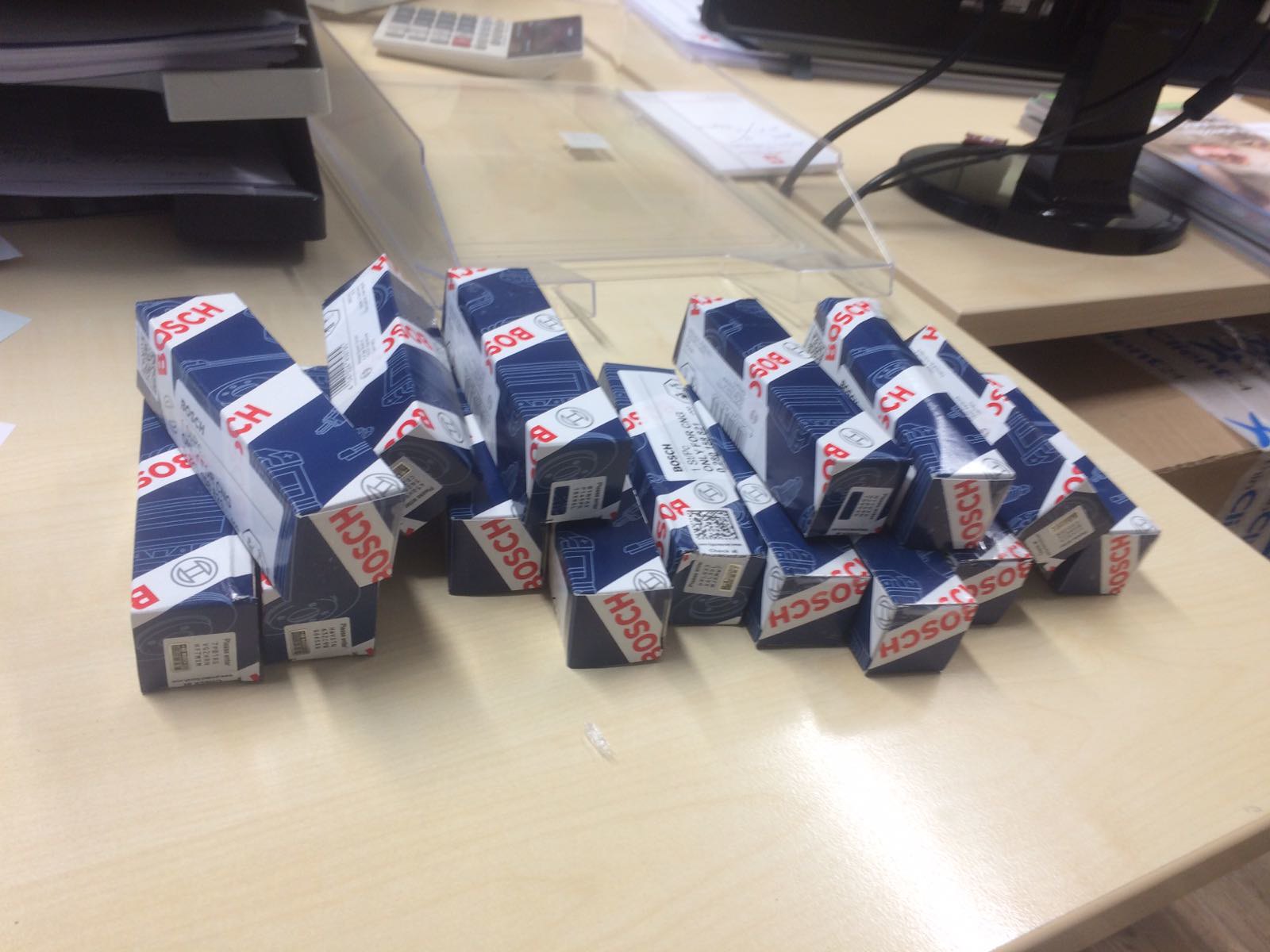This photograph captures a cluttered desk area with several office supplies and equipment. In the upper right-hand corner, there is the base of a black computer monitor with a black cord dangling through a hole in the desk. Nearby, a white calculator is visible towards the upper left. Dominating the center of the image are several blue rectangular boxes with white labels and red "Bosch" lettering; these boxes appear to be stacked both vertically and horizontally and feature barcodes and stickers on some ends. Additionally, there is a noticeable stack of black books lying on top of one another on the left side of the desk. A cardboard box with a white label and blue writing is also present on the right-hand side. The desk itself is a light wooden brown, adding warmth to an otherwise utilitarian scene.